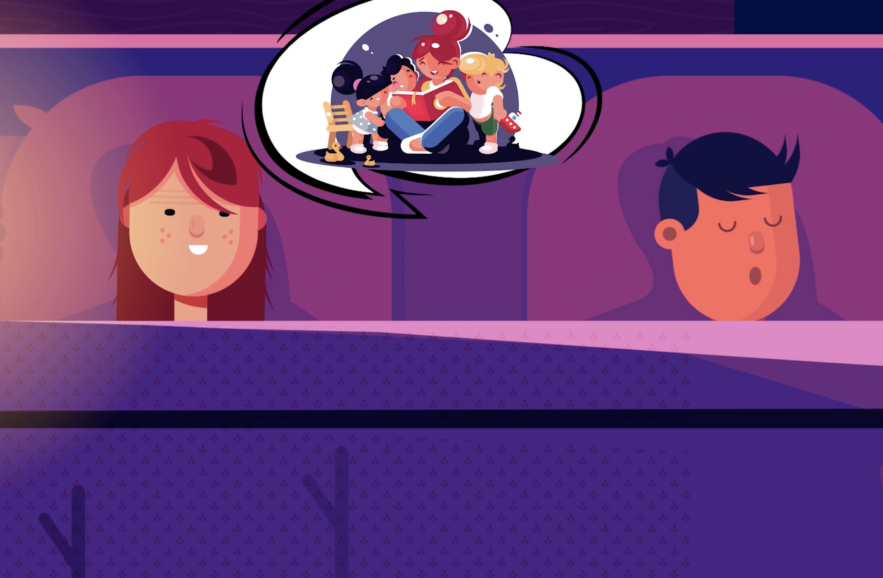The image is a vibrant and clear multi-color digital piece in a square format, depicting a scene that blends indoor and outdoor elements seamlessly. At the center, two people are lying in bed; the woman, positioned on the left, and the man on the right. They are enveloped in a purple blanket that features a prominent vertical black line towards the bottom. The man is fast asleep, evidenced by his closed eyes and open mouth, whereas the woman is awake, exhibiting a small, serene smile. 

She has brown hair and freckles, adding to her detailed appearance. Above her head, a thought bubble reveals her imagination: a scene where she is joyfully reading a book to three children— two with dark hair and one with blonde hair. She is depicted sitting with her legs crossed, holding a book, with the children gathered around her, all engaged. 

Additionally, the image includes two 'Y' shapes situated in the lower center and lower left corner. Despite multiple elements in the scene, the background is non-definitive, giving the image a surreal, dream-like quality suitable for the imaginative thought bubble. The overall setting is bright and clear, with a notable absence of words or numbers, enhancing the visual storytelling.